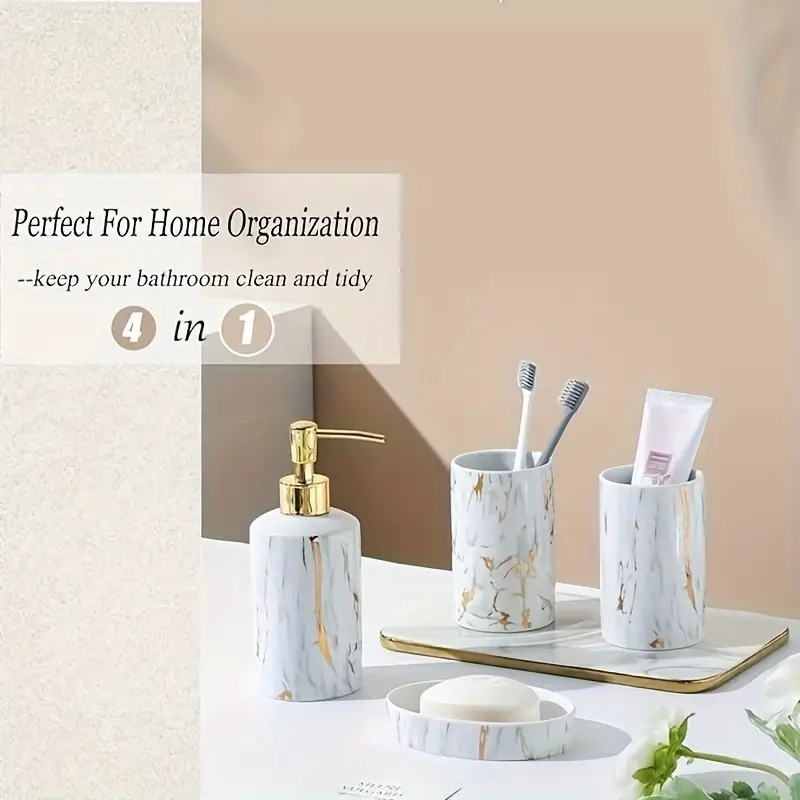The image captures a neatly organized bathroom countertop, aligning with the message "perfect for home organization" and the smaller caption "keep your bathroom clean and tidy." The vertical photograph showcases a cohesive set of four bathroom essentials, all adorned in a white and gold marble pattern. Centered on the white countertop are two cylindrical holders; the one on the left cradles two toothbrushes, while the right one contains a tube of toothpaste. Accompanying these are a matching soap dispenser and a soap dish holding a white bar of soap. The text overlay details the four-in-one organization solution, with the number four highlighted in a dark tan circle, followed by the word "in" in italicized cursive, and the number one in a light tan circle. The entire setup epitomizes elegance and functionality, perfect for maintaining a tidy bathroom space.